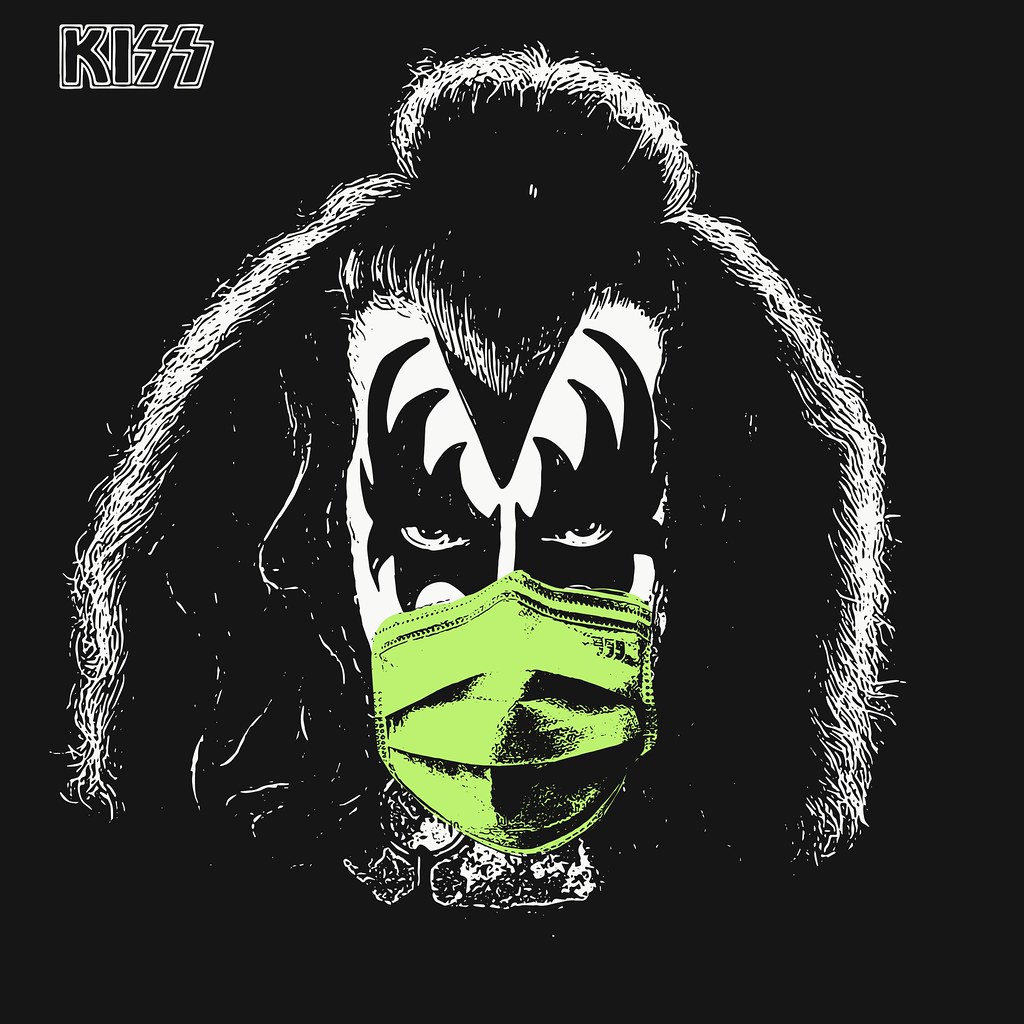The image is an album cover from the band KISS, featuring Gene Simmons, one of its iconic members. Positioned in the upper left corner of the cover is the band's name "KISS" written in a double white outline. The image is primarily black and white, highlighting Simmons in his trademark "Demon" persona from the late '70s and early '80s. His face is painted white with dramatic black spikes extending above and below his eyes, which are dark and menacing. His hair is black with white streaks, styled to a point above his eyebrows and cascading around his face, resting just above his shoulders. Adding a curious twist to the image, Simmons is wearing a light green surgical mask with an indistinct insignia that appears as three small commas on the right-hand side above his mouth. This mask stands out vividly as the only colored element in the otherwise monochrome composition, contributing to the dark and edgy yet somewhat parodic aesthetic typical of a KISS album cover.